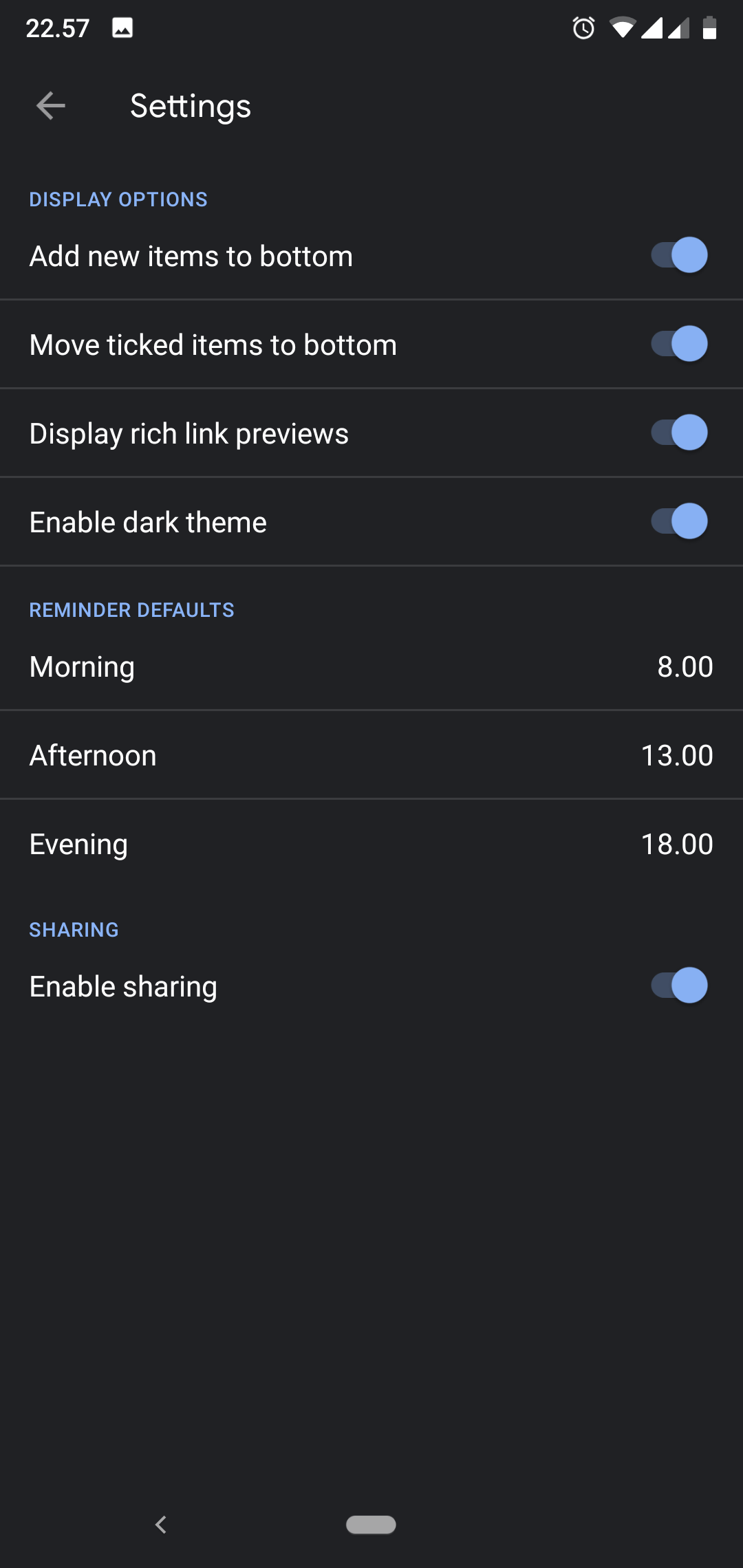Screenshot of Mobile App Settings Menu

At the top of the mobile screenshot, the current time (22:57) is displayed in white font alongside a white mountain icon. On the upper right, various status icons are shown, including an alarm clock, Wi-Fi, mobile data, and a half-filled battery indicator.

Below the status bar, a gray back arrow pointing left is accompanied by the word "Settings" in white. The settings are organized under three main headings in blue: "Display Options," "Reminder Defaults," and "Sharing."

Under "Display Options," there are four settings listed in white text:
1. Add new items to the bottom
2. Move ticked items to bottom
3. Display rich links preview
4. Enable dark theme

Each of these settings has a corresponding toggle switch on the right side, all of which are turned on and highlighted in blue.

The next section, "Reminder Defaults," displays default times for reminders in white text:
- Morning: 08:00
- Afternoon: 13:00
- Evening: 18:00

The final section, "Sharing," includes a single option:
- Enable sharing, with its toggle switch also turned on and highlighted in blue.

The entire interface is displayed with a black background, indicating that the dark theme is enabled.